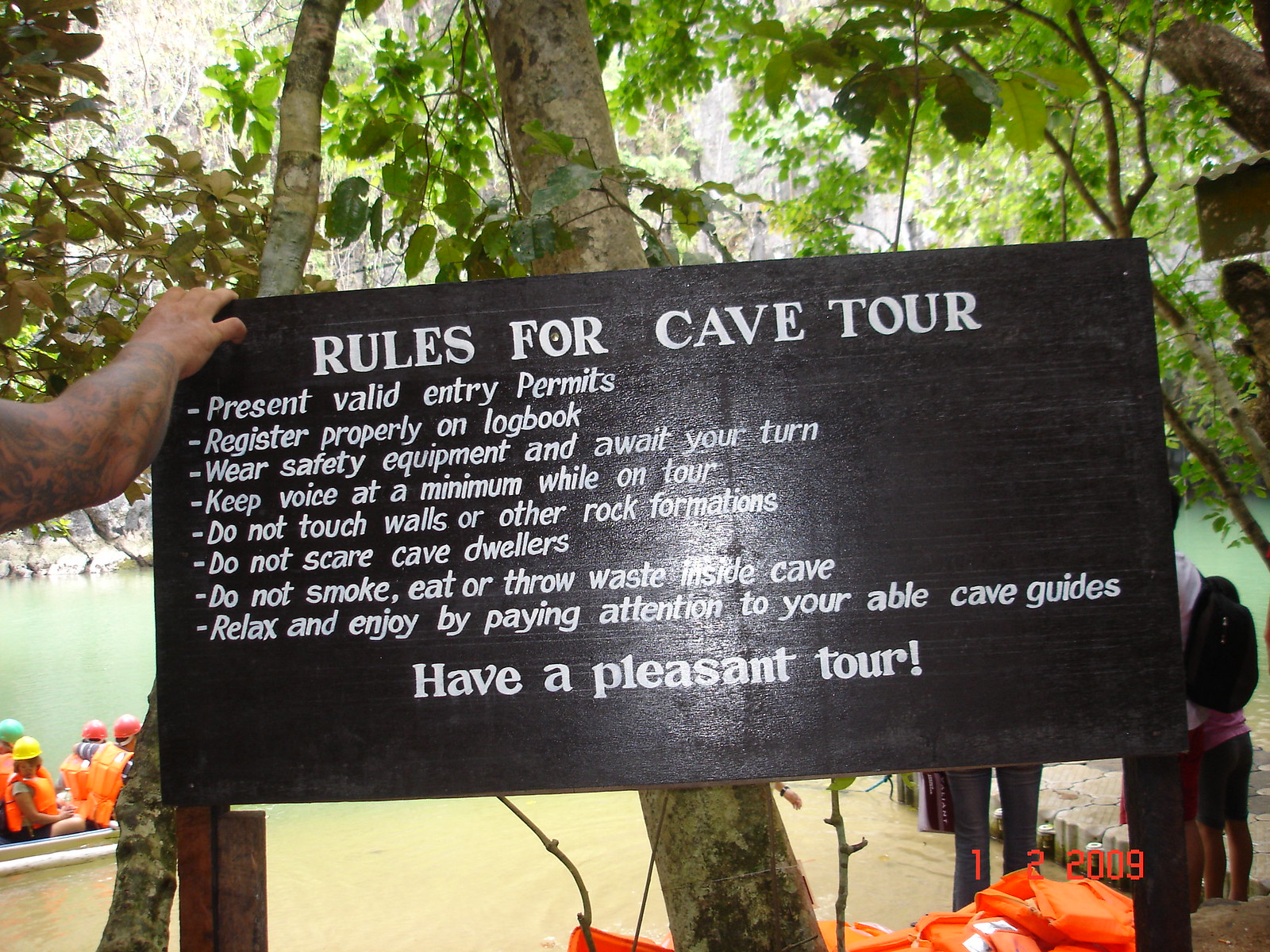A black wooden sign with white lettering, titled "Rules for Cave Tour," is prominently displayed on a tree. An arm reaches out to hold the top left corner of the sign. The rules listed include: present valid entry permits, register properly on the logbook, wear safety equipment and await your turn, keep voices at a minimum while on tour, do not touch walls or other rock formations, do not scare cave dwellers, do not smoke, eat, or throw waste inside the cave, and relax and enjoy by paying attention to your able cave guides. The sign concludes with "Have a pleasant tour," and a date noted at the bottom as 1209. In the background, a body of water transitions from light green to brown, where several people wearing helmets and orange life vests navigate a canoe or raft. Further beyond, tree branches with green leaves are visible, adding to the scenic setting. On the bottom right corner under the sign, a stack of orange life jackets can be seen, suggesting a boat tour through the cave.